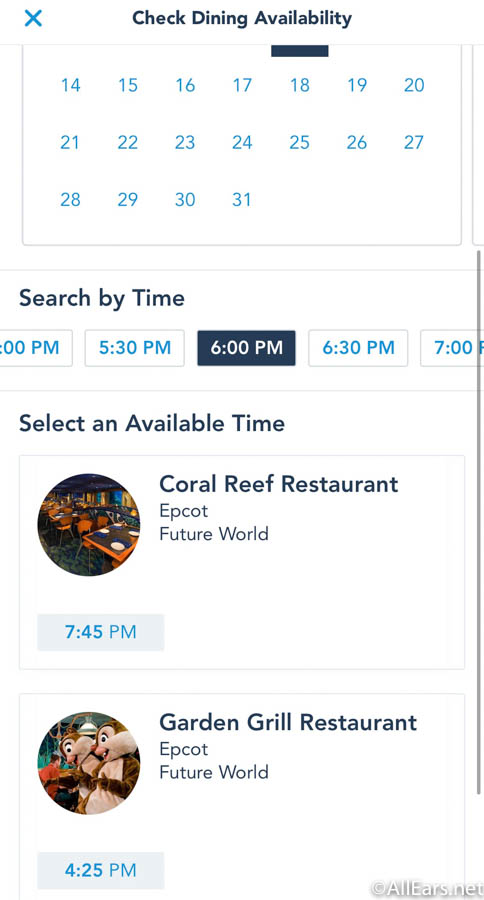Here's a detailed, cleaned-up caption:

---

The image depicts a screenshot from a reservation app, seemingly used to book dining reservations. At the top of the screen, there's a header labeled "Check Dining Availability." Beneath this header, there is a calendar display. Each date is prominently marked in blue to stand out against the white background of the interface. Below the calendar, a "Search by Time" section lists different time slots, starting from 5 p.m., with options progressing in 30-minute increments: 5:00 p.m., 5:30 p.m., 6:00 p.m., 6:30 p.m., and 7:00 p.m. The selected time slot, 6:00 p.m., is highlighted in a dark blue box, distinguishing it from the other options that are highlighted in light blue.

Further down, the screen displays available reservations for two restaurants. The first option is "Coral Reef Restaurant" located in "EPCOT, Future World," with an available time at 7:45 p.m. This option is accompanied by a thumbnail image of the restaurant on the left. The second option is "Gordon Grove Restaurant," also situated in "EPCOT, Future World," with an available reservation time at 4:25 p.m.

---

This caption provides a comprehensive and organized description of the screenshot, making it easier to understand the details presented in the image.